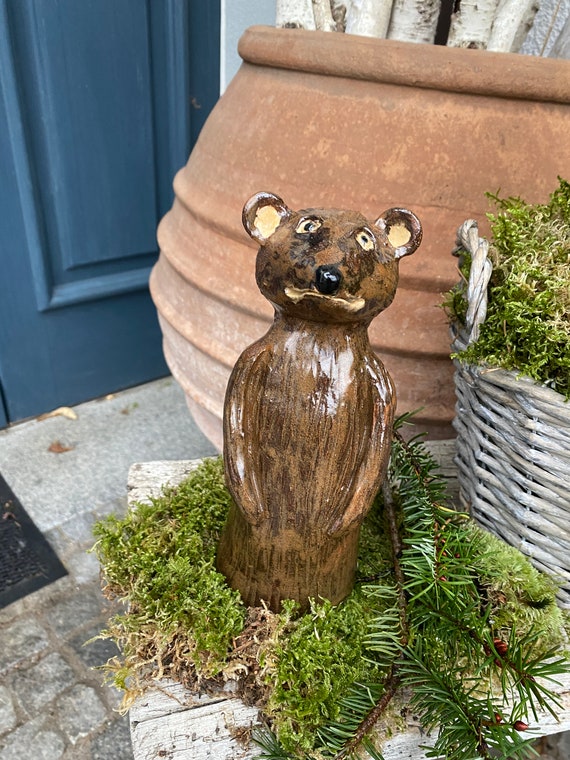This outdoor photograph, taken during the daytime, features a whimsical ceramic bear statue placed near a front door. The bear, approximately 16 inches tall and seemingly crafted from clay, has a long, narrow brown body with noodle-shaped arms resting at its sides, lacking defined fingers or paws. Its round head features a black nose, black-dotted eyes, and a mouth carved in a flat line, all highlighted with light brown and tan accents. The bear's ears also protrude with light yellow interiors. Nestled in a decorative bed of green moss and pine needles, the statue is positioned in front of a large terracotta pot filled with white firewood and next to a white wicker basket with additional moss or plants growing inside. To the left, a blue door with a black doormat below it adds to the charming, rustic outdoor setting.